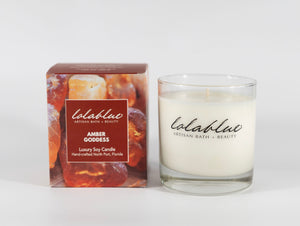The image features a luxurious white candle housed in a clear glass container, inscribed with stylized, cursive black text that reads "Lala Blue." The text is somewhat difficult to decipher due to its intricate design. Below this, in very small font, there is additional writing that is nearly impossible to read. Accompanying the candle is its packaging—a predominantly brown-toned box with lighter brown and tan accents. The box displays images that are unclear but resemble baked bread or warm coals. Central on the box is a brown label with cursive writing in white that mirrors the "Lala Blue" text on the candle. The label also prominently features the phrase "Amber Goodness," indicating the candle's scent. Both the candle and its box appear to be of high quality, making them an excellent gift choice. The background of the image is primarily white with subtle hints of gray.